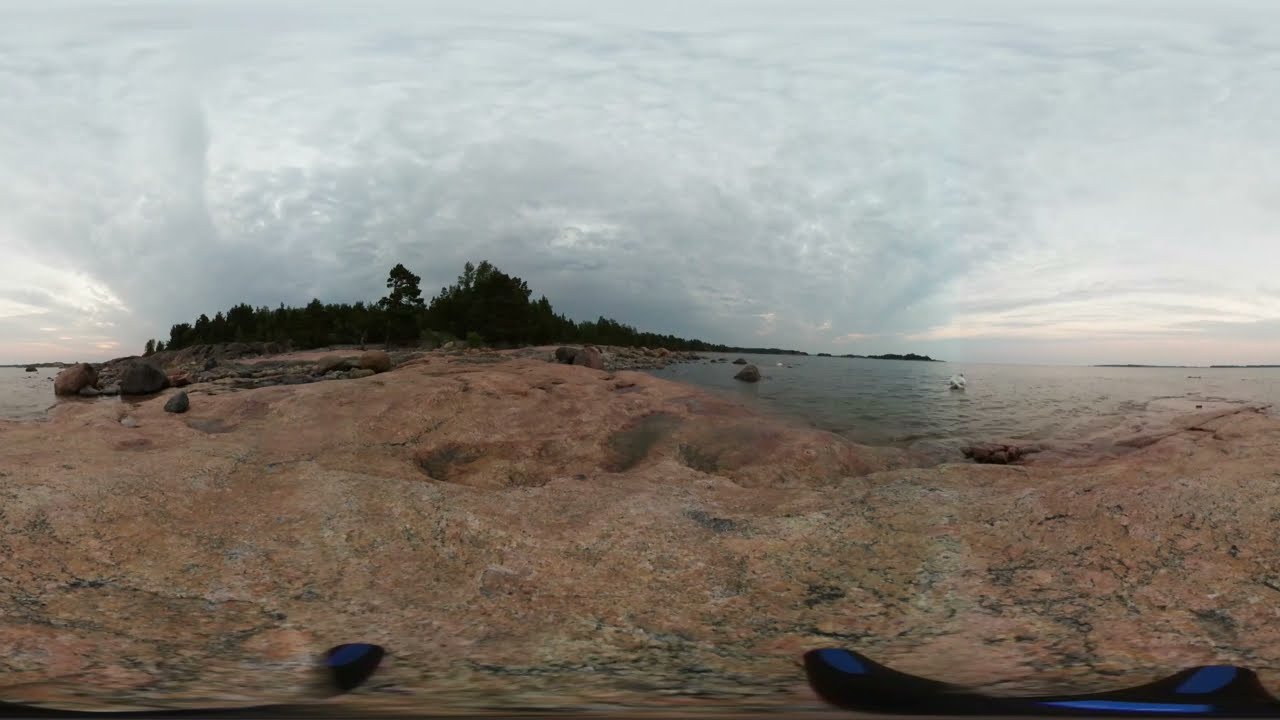This image captures a dramatic outdoor landscape, seemingly distorted as if taken through a fisheye lens. Dominating the foreground is a wavy, hilly expanse of rocky terrain, characterized by its rugged texture and a palette of tan, copper, and brown hues interspersed with darker shades. Large boulders are sporadically scattered throughout this area. To the right, an expansive gray body of water is visible, fringed by rock formations that extend into its expanse. Above, a vibrant blue sky is dotted with numerous fluffy clouds, some of which have white streaks extending outward. In the distance, clusters of dark green pine trees and other foliage create a dense, lively canopy. The entire scene is bathed in daylight, emphasizing the natural colors and textures of this unique outdoor setting.